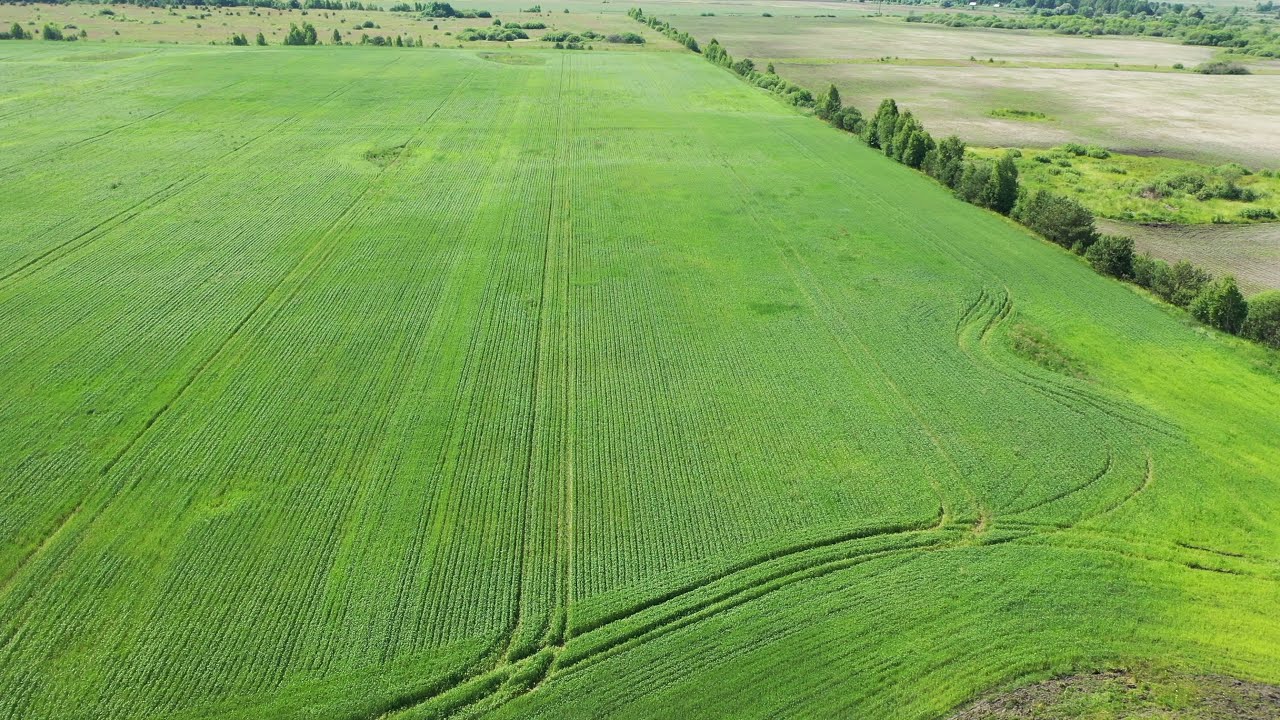The image showcases a vast expanse of green farmland, occupying around three-quarters of the frame, with well-defined tracks running through the crops, likely from tractors or combines. The field is a verdant green, indicating well-maintained crops, and is bordered by a strip of dirt or undeveloped land, which appears lighter in color. This area features scattered trees and shrubs, creating a natural barrier between the farmland and the lighter, possibly barren area. In the upper right corner and stretching into the far background, a dense line of trees and more scattered shrubbery can be seen. The hues in the image span various shades of green, interspersed with browns, grays, and blacks, suggesting different stages of growth and soil conditions. The overall impression is a serene, expansive outdoor scene dominated by agricultural elements with no text visible.